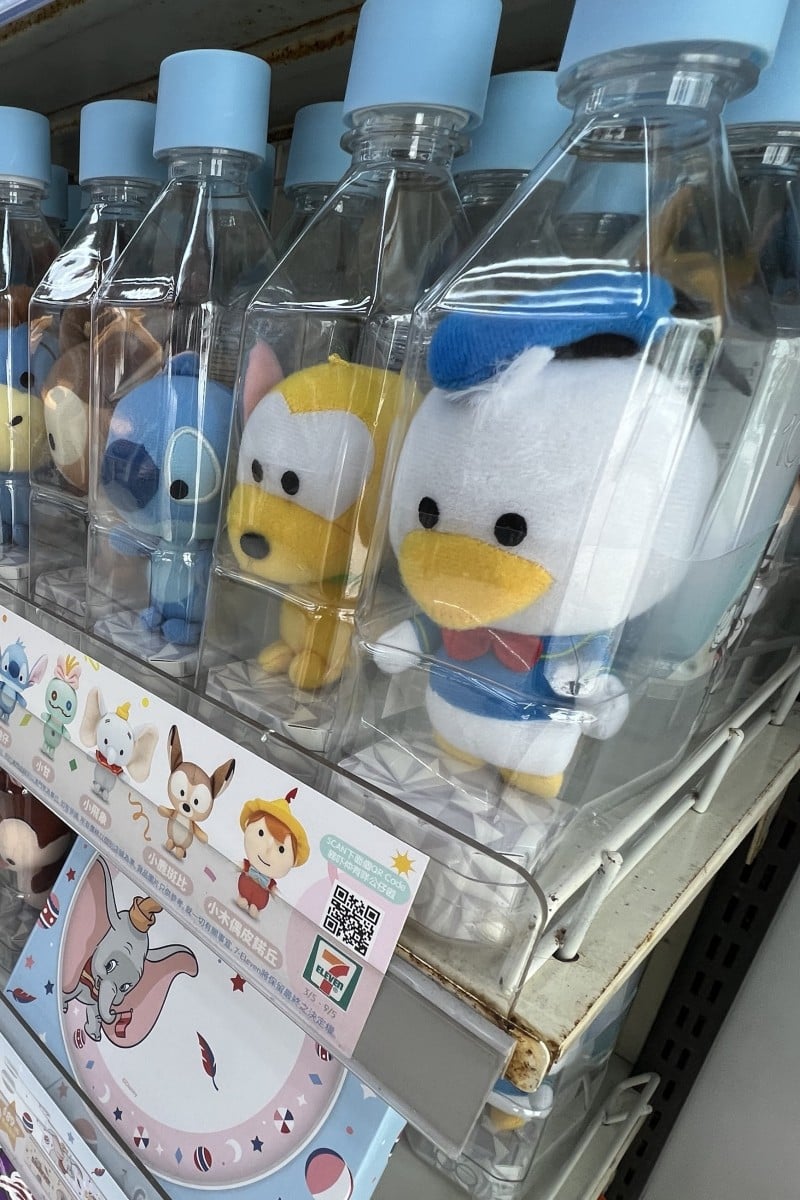This is a vertical, close-up photograph of a store shelf display at a 7-Eleven, featuring stuffed Disney characters enclosed in clear, tall, shiny plastic bottles with large blue screw caps. The containers are arranged vertically, standing on shelves, and each bottle contains a different character. The focal point is a bottle with a stuffed Donald Duck, which has a white round head, a short yellow beak, two circular eyes, a blue hat, a red bow tie, a blue top, white pants, and little yellow feet. To its left is a bottle with Pluto, the light brown dog with a large white area around the eyes and two small circles for pupils. To the left of Pluto is a bottle with Stitch, Eeyore follows, and there are additional characters like Pinocchio, Bambi, and Dumbo in similar containers. Below these bottles on the shelf is a label featuring animated images of the characters and Japanese lettering, including the 7-Eleven logo and a QR code. On the lower shelf to the left is a plate with an image of Dumbo.